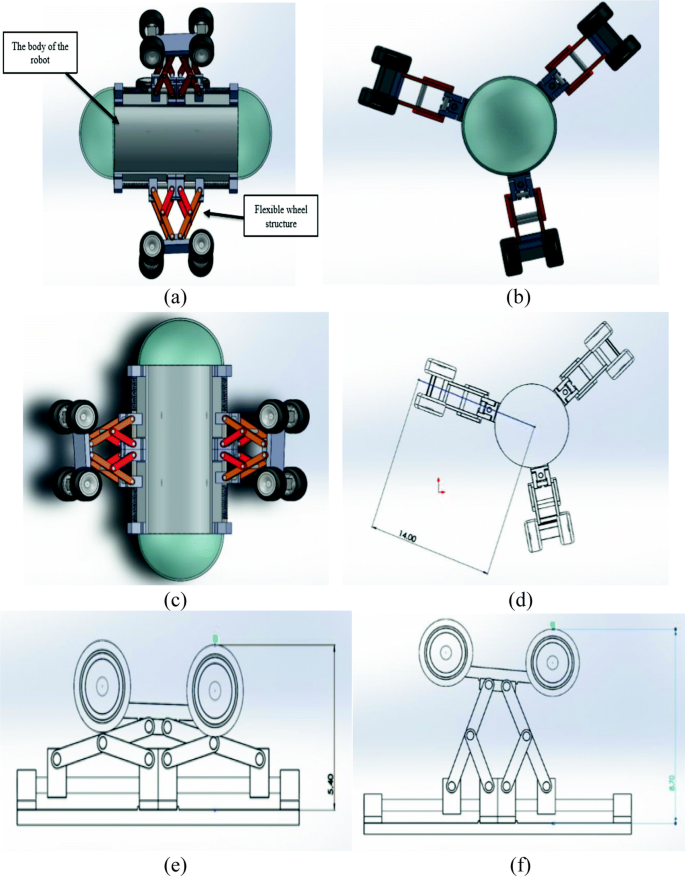The image is a detailed graphic illustration consisting of six panels, labeled A through F, arranged in two rows of three. The first three panels (A, B, C) display color graphics in shades of green, silver, red, and black, while the last three panels (D, E, F) feature black and white technical drawings.

Panel A, labeled "Figure A," provides a side view of a cylindrical robot, which is colored gray with green tips. It has eight wheels on either side and is annotated with captions pointing to the "body of the robot" and "flexible wheel structure." 

Panel B, labeled "Figure B," shows an overhead view of the robot, revealing the green tip and the six wheels extending outward from the robot's center akin to radiating arms.

Panel C, labeled "Figure C," depicts the robot in a vertical layout, again showing its eight wheels with four on each side. Similar to the previous views, the robot features gray and green coloring.

Panel D, labeled "Figure D," mirrors the overhead layout of Panel B but in a black and white drawing style, including a dimension labeled 14.00.

Panels E and F are technical drawings of the robot’s flexible wheel mechanisms. Panel E shows the accordion-like pantograph structure minimally extended, while Panel F depicts it fully extended, elevating the wheels significantly off the ground.

The entire image, which is vertically rectangular without any overall border, adopts a modern graphic style to illustrate the design and functionality of a cylindrical robot that could be used in industrial settings to transport items.